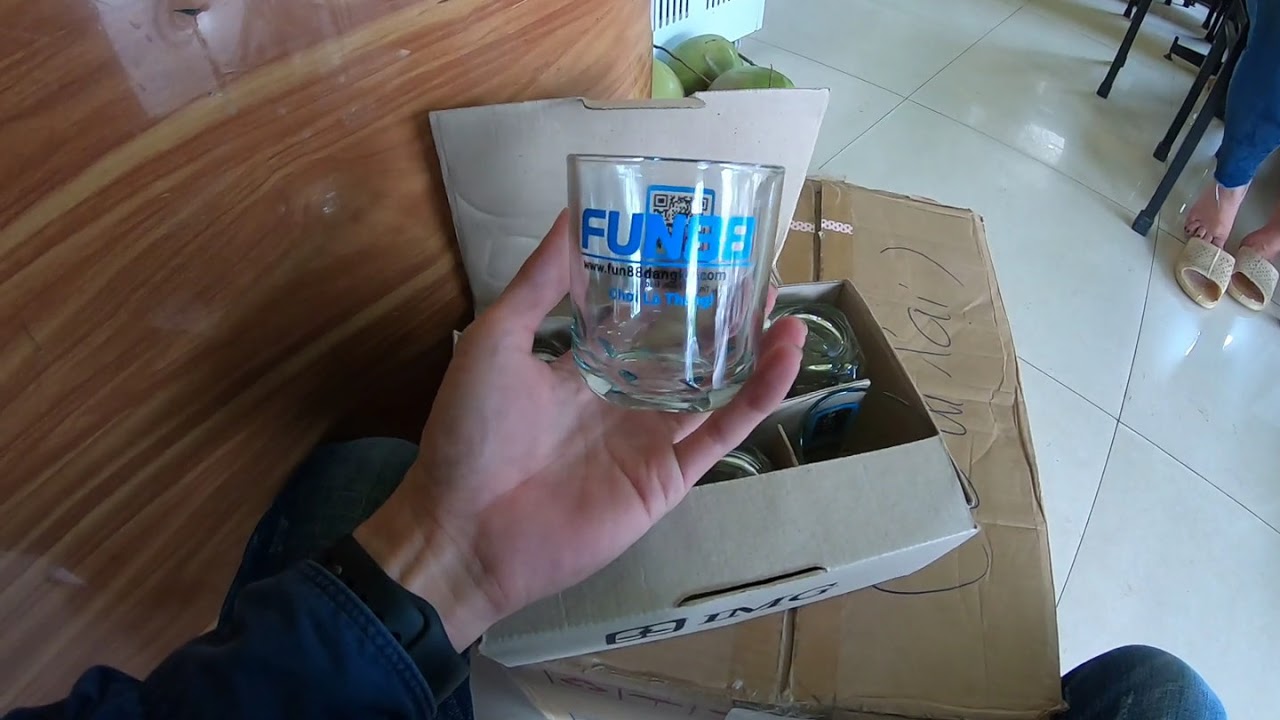The image depicts a white man seated on a white tiled floor, with blue jeans covering both his knees. His left hand, clad in a dark blue sleeve, holds a clear glass featuring blue text "F-U-N-E-E" along with some other illegible writing and a website URL "WWW.FUN88DANG...". This glass appears to have come from a larger cardboard box resting on his lap. The box is brown with a dark strip down the middle where it opens, and it has some unreadable writing on it. Inside this box, there's another silver-colored box, which partially obscures a barcode visible through the glass. In the upper right corner of the image, a woman’s feet, possibly in blue jeans, are visible; her feet are out of her sandals. The background features a wooden or wood-grain wall on the left side. Additionally, light green circular objects are spotted on the floor beyond the flaps of the box.